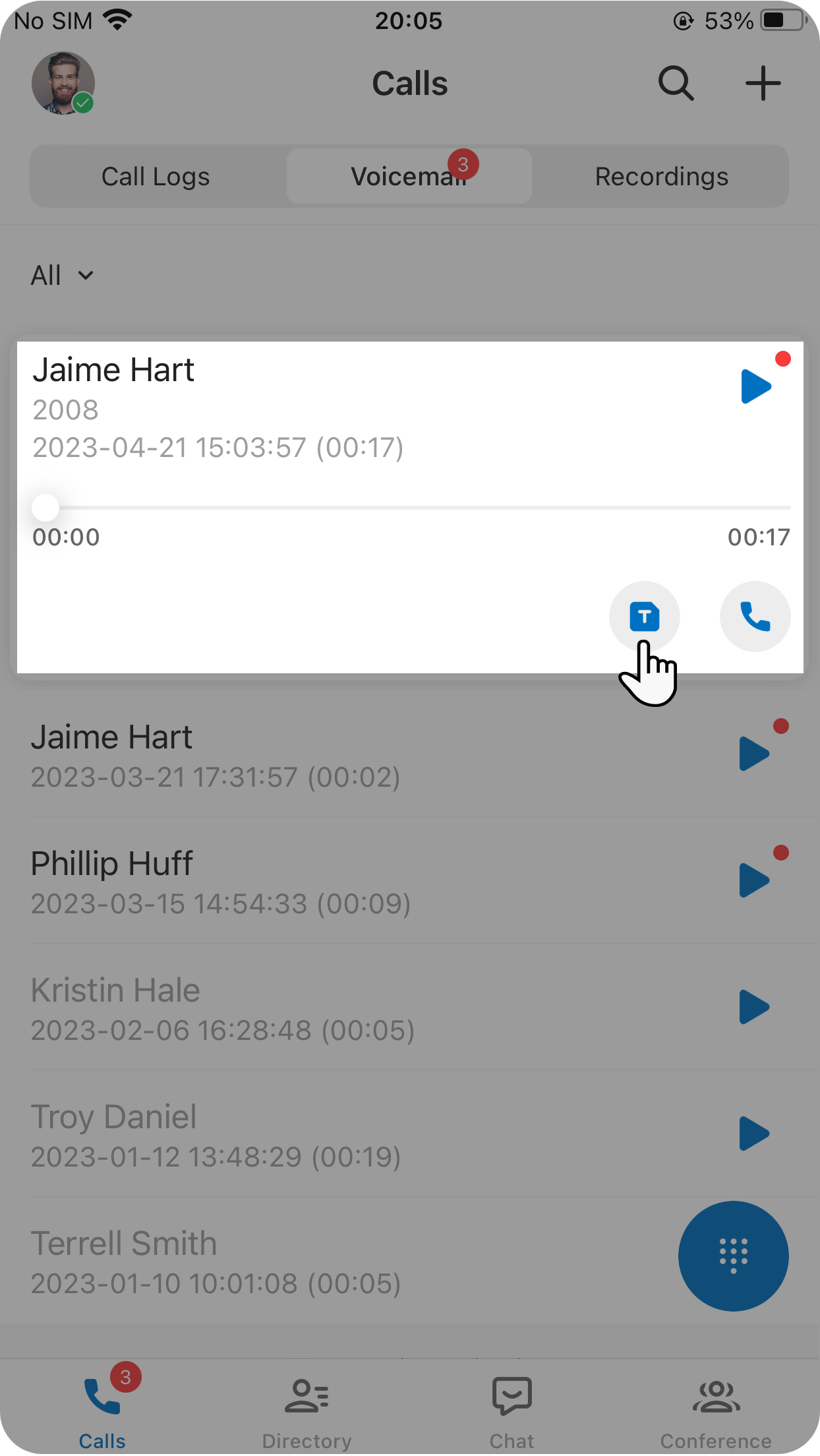The detailed caption for the image could be:

"This is an edited screenshot of a cell phone's call logs section, featuring a clean white background. At the top center, 'Calls' is prominently displayed in large black letters. Positioned just beneath this header are three tabs: 'Call Logs,' 'Voicemail,' and 'Recordings,' with 'Voicemail' currently selected. A red notification circle above the word 'Voicemail' indicates the presence of a new voicemail.

Below this, a pop-up box displays detailed information about the voicemail. In the top left corner of the box, the caller’s name is visible, followed by the date and time of the voicemail. A slider bar occupies the center, allowing the user to fast-forward or rewind the message. In the top right corner of this pop-up, there is a play button, and directly above it, a red dot signifies that the message has not been listened to yet.

At the bottom of the pop-up box, there is an icon featuring a white 'T' on a blue piece of paper, symbolizing the transcript option. An edited mouse pointer is directed at this icon, illustrating that selecting this option will transcribe the voicemail message. This screenshot serves as an instructional guide on how to access voicemail transcription on the device."